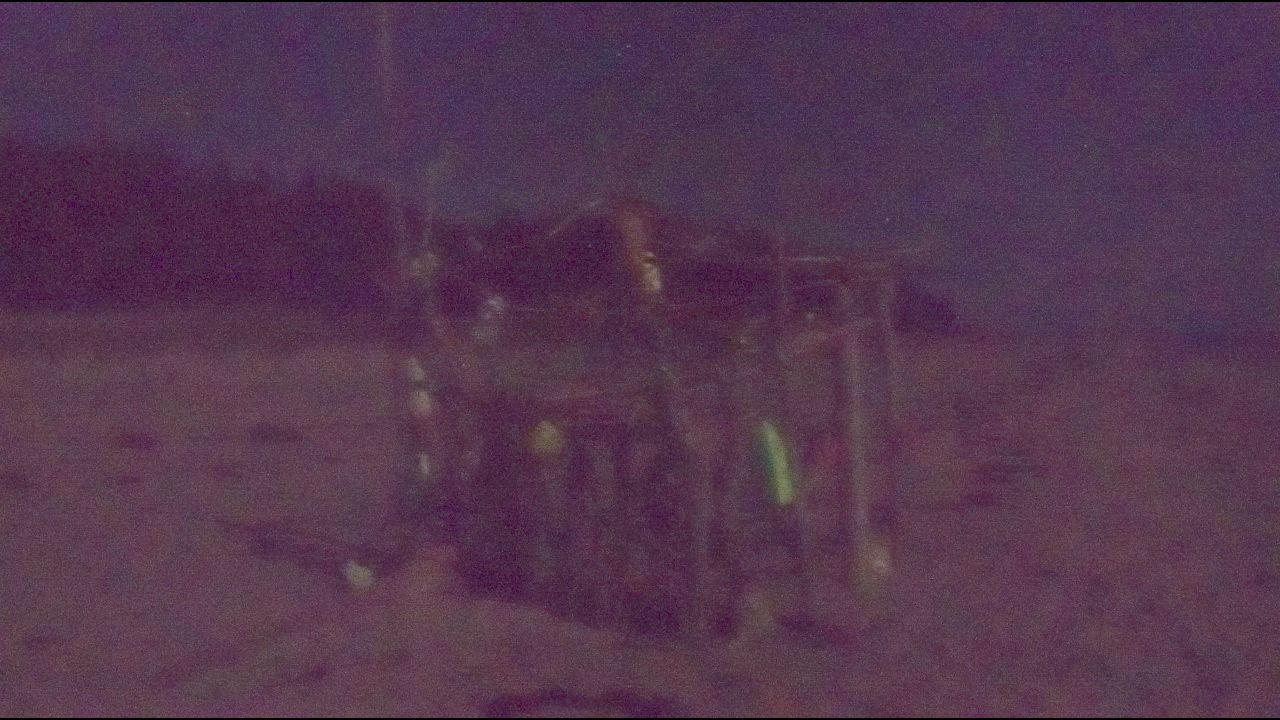The image is very dark and blurry, featuring a dirt ground and a lighter sky in the background with varying shades of purple. A line of trees or possibly a mountain runs along the horizon. The central focus of the image is a box-like, unclear object with numerous pipes or sticks sticking out of the ground, forming an irregular framework. A small, green vertical mark can be seen on the bottom right side of this structure. The overall impression is highly confusing and resembles a possibly impressionistic depiction, making it difficult to accurately identify the elements present.